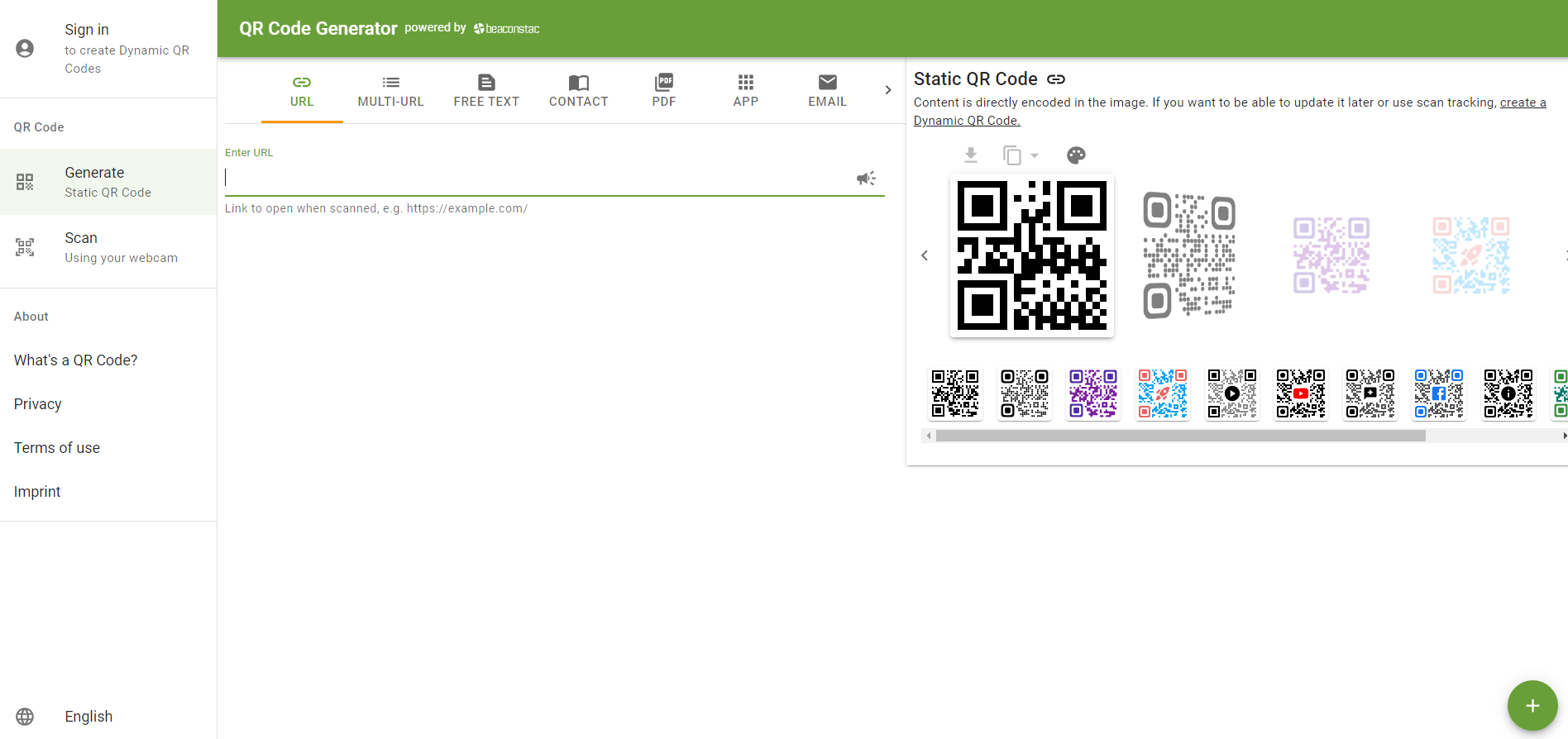This web page features a clean, white background with a prominent green banner extending across the top from a few inches left of center to the far right. On the left side of the green banner, text in white reads "QR Code Generator powered by [something]." Below the banner, aligned to the left column, there is an icon of a head and shoulders with the instruction "Sign in to create dynamic QR codes" written in dark ink. 

Further down the page, underneath the instructional text, there is a light blue box containing more information about QR codes. This section includes a menu with options listed in white text: "Generate Static QR Code," "Scan using your webcam," "About," "What's a QR code?", "Privacy," "Terms of Use," and "Imprint." At the very bottom of the page, a globe icon is situated next to the word "English," indicating the language setting.

In the central area, there is another column with a header in white text that says "URL," underlined by an orange line and highlighted in green. Adjacent to this, a series of menu items spans from left to right, each with an accompanying symbol: "Multi URL," "Free Text," "Contact," "PDF," "App," and "Email." These items help users select the type of QR code they want to generate.

Beneath the menu options, a prompt reads "Enter URL," accompanied by a text input field where users can type their desired URL. To the middle-right section of the page, there is another box outlined in light blue or gray, titled "Static QR Code." This box contains numerous watercolor QR code designs, showcasing different styles available for static QR codes.